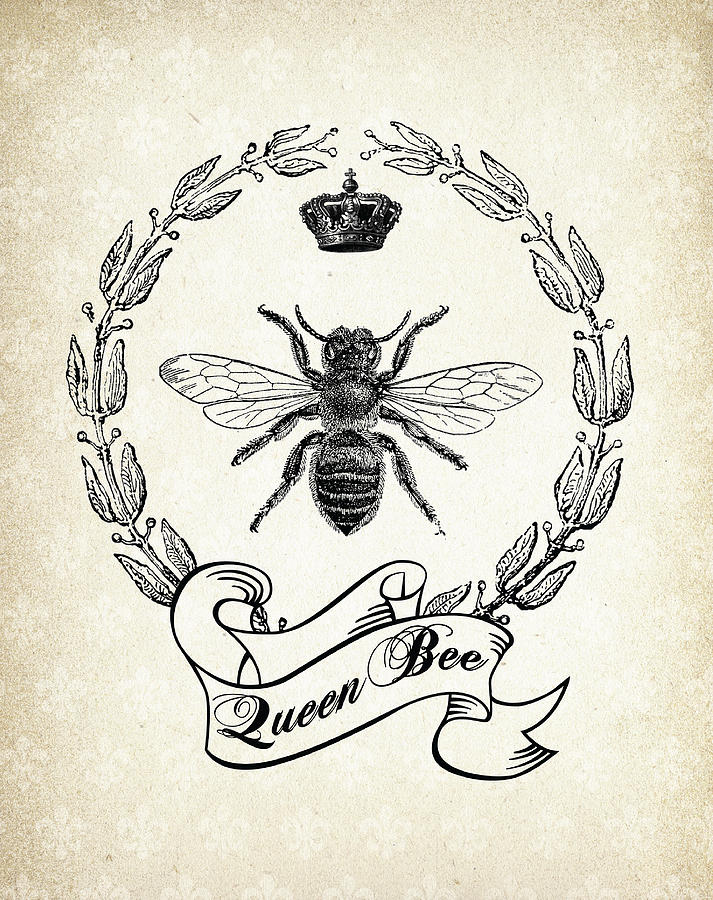The image features a meticulously outlined drawing set against a subtly textured, cream-colored background adorned with repetitive fleur-de-lis patterns. Centrally positioned is a large, intricately detailed bee, evoking the precise illustration style found in old field guide textbooks. The bee, complete with two pairs of wings, antennae, six legs, and a striped abdomen, is rendered in black and white, suggesting the use of pencil or pen. Above the bee, a finely detailed crown is situated, resembling an ornate clip-art representation of a royal crown. Enveloping the central elements is a circular crest formed by laurel leaves, which converge near the top where the crown sits. Below the bee, a traditional tattoo-style banner stretches across, inscribed with the words "Queen Bee" in elegant cursive. The overall composition is evocative of a potential tattoo design, marrying classic emblematic elements with a timeless, monochromatic palette.